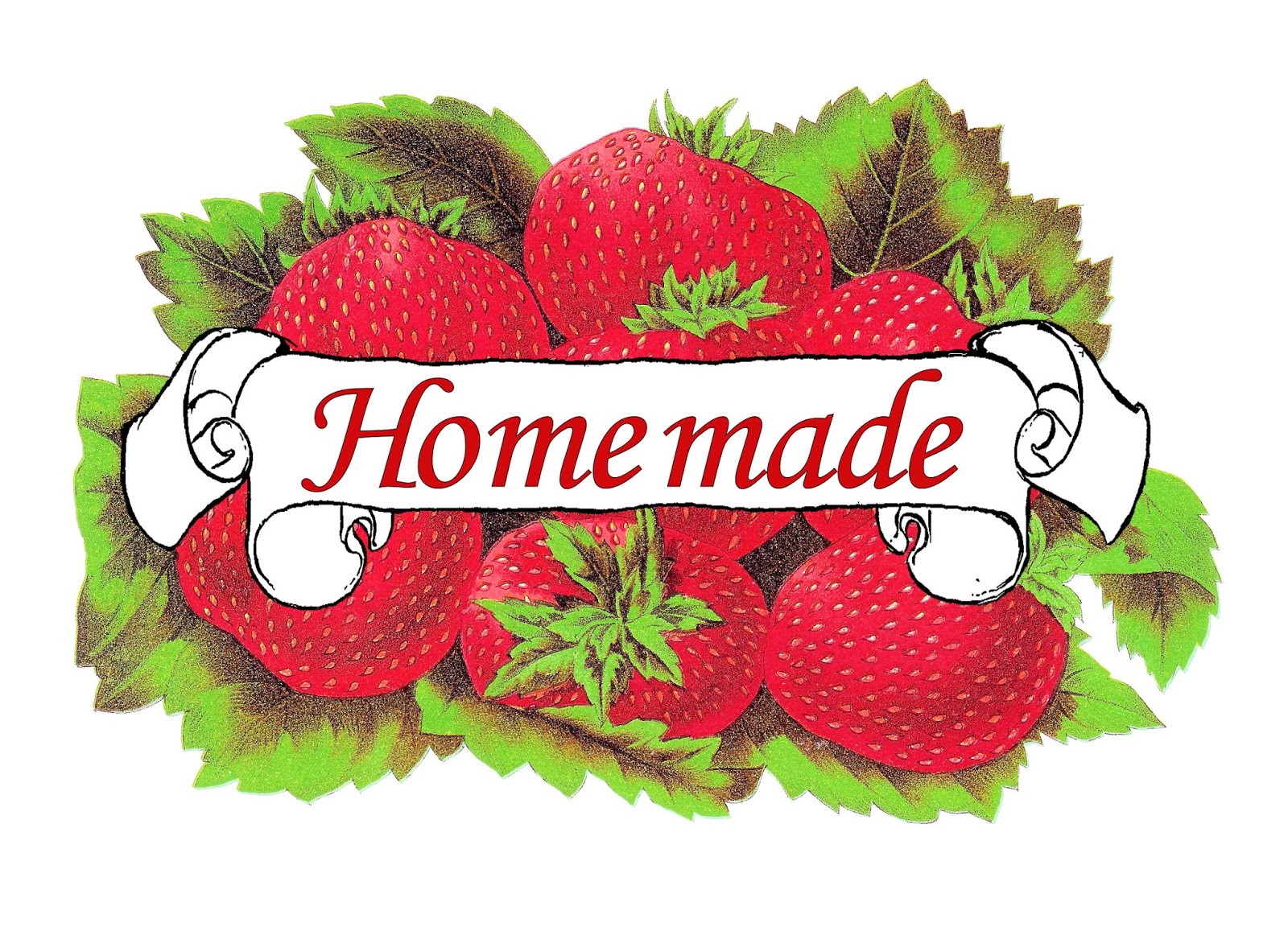This image features a marketing-style graphic designed to resemble a logo or a label, ideal for a homemade product. Prominently set against a white background with no external border, the focal point is a white banner with a black border and scroll design at each end. In the center of the banner, the phrase "Home Made" is inscribed in a striking red serif font, italicized, with only the letter H capitalized. Surrounding the banner is a lush arrangement of vibrant red strawberries, numbering around eight or nine, each illustrated with bright red circles and speckled with tiny yellow seeds. The strawberries, complete with their bright green leafy tops, rest on a bed of large green leaves, which frame and accentuate the fruit. This visually appealing and detailed graphic could easily serve as a charming label for homemade goods, such as jam jars, emphasizing both freshness and artisanal quality.